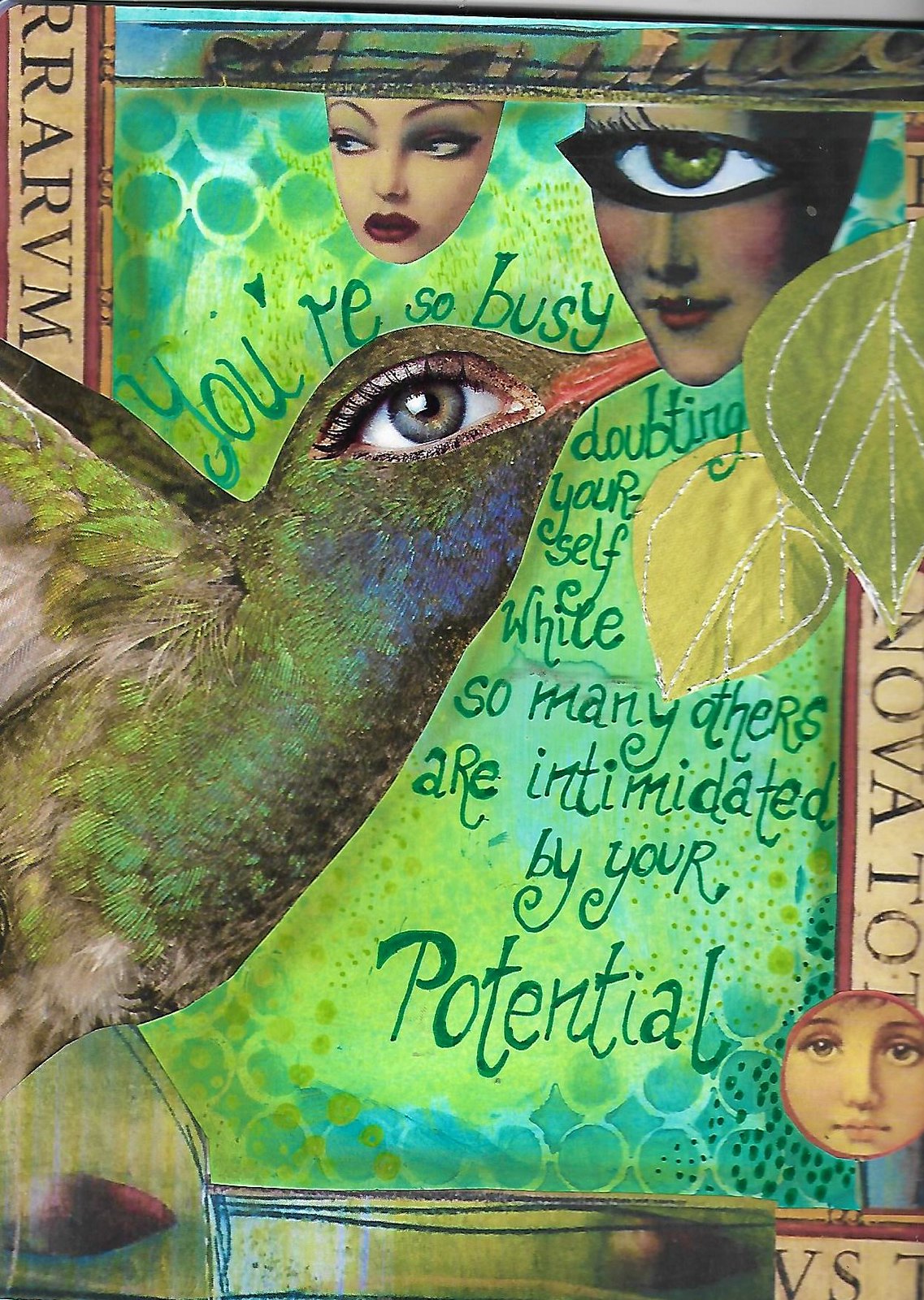The image depicts an abstract piece of art that combines surreal elements with vibrant colors and text. Dominating the composition is a green hummingbird, notable for its unusually large human eye. The bird’s orange beak is strikingly piercing a human face that possesses a single enormous eye, which spans almost the entire width of the face. Adjacent to this face, on the left, is another face with two regular eyes and red lips, lacking a body just like the face being pierced by the hummingbird. The background of the piece is filled with circular patterns in varying shades of green, adding to the surreal quality. Positioned towards the bottom right corner is a circular image resembling a child’s face drawn in a simplistic manner. Green text, elegantly integrated into the artwork, conveys the motivational message: "You're so busy doubting yourself while so many others are intimidated by your potential." Additionally, black text appears rotated 90 degrees clockwise on the top left, partially cut off, reading "R-R-A-R-V-M."